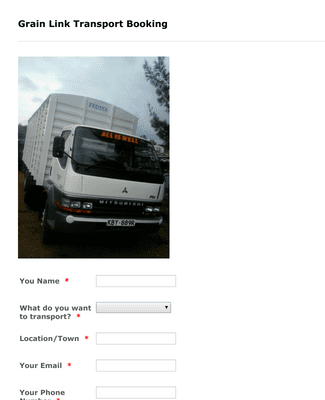The image is a screenshot of a webpage for Green Link Transport Booking. At the top, there is a bold black header that reads "Green Link Transport Booking." Below the header, there's an image of a predominantly white transport truck featuring some black details. The brand of the truck appears to be Mitsubishi, and the side of the truck displays the phrase "All is Well" at the top. The truck's license plate starts with the letter 'K.' The overall ambiance of the image is rather gloomy, suggesting overcast skies or diffused lighting, indicating it's not a sunny day.

Beneath the truck image, the webpage provides various fields to fill in user information, including name, transport item details, location in town, email, and phone number. These fields are likely to be used for initiating contact between the user and the transport company to coordinate the booking details. The screenshot only showcases one type of transport truck, prompting potential questions regarding the availability of various truck options catered to different transport needs.